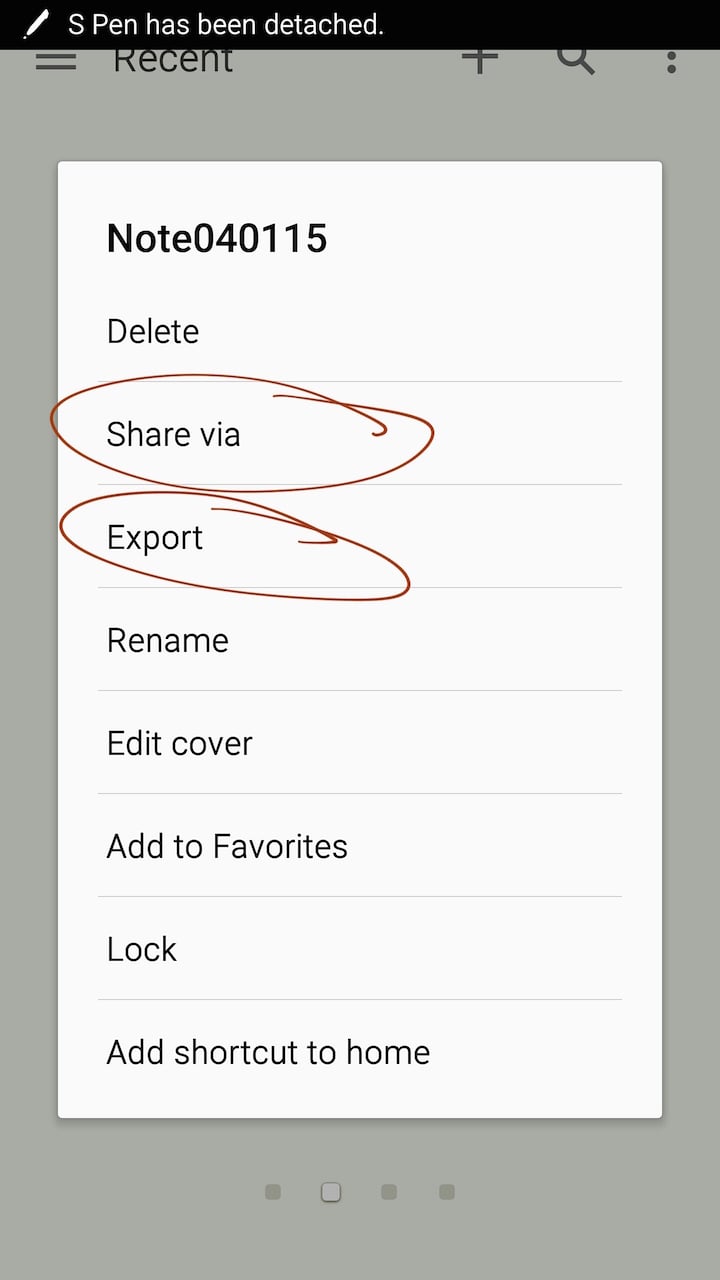The image showcases the top layer of an interface with a gray background. A black pen is depicted, although it has been detached from its top part. At the top, there's text displaying the letter "S," and a magnifying glass icon is visible in the hamburger menu. The bottom features a series of elements: a dot followed by a set of three squares. In the middle of the image, a white menu is prominent, with several options listed. The top section of the menu reads "note 040115" and includes a "delete" option. Further down, there are additional functions like "align," "share view," depicted as a red circle with align options, "export," "rename," "edit," "cover," "add to favorites," "lock," and "add shortcut to home." The overall scene is set against a gray background.